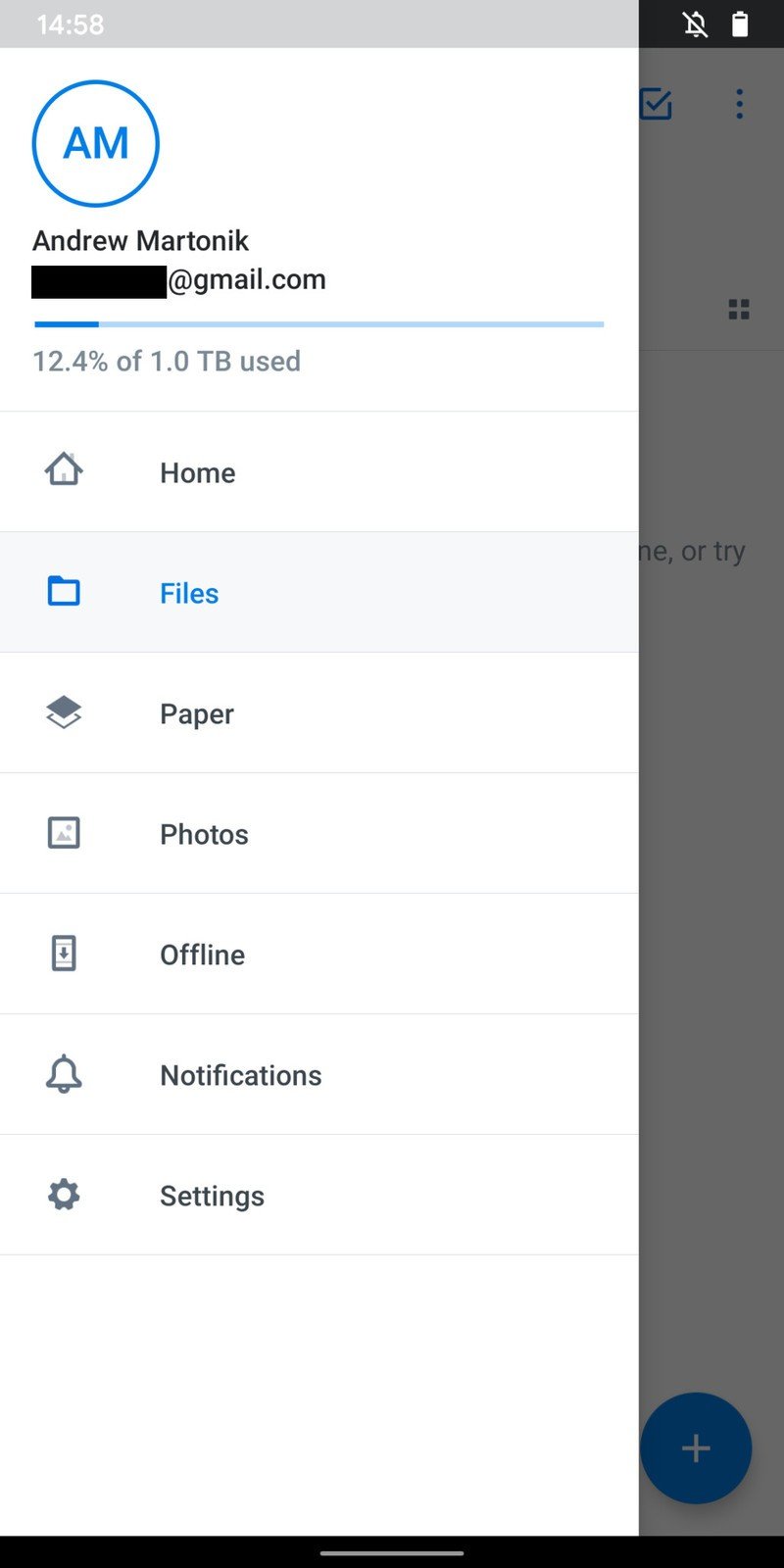The image, captured on a mobile device, shows the user interface of an email account. At the very top of the screen, a gray bar displays the time as 14:58, situated in the top left-hand corner. The main portion of the image features a vertical white rectangle. Prominently, there is a circular icon with the letters "AM" in blue, surrounded by a white circle with a blue border. This icon represents the user Andrew Martonik, with his name clearly spelled out beneath it.

Andrew's email address is partially obscured by a black horizontal bar, masking the first part, but it is apparent that the domain is @gmail.com. Additionally, the image indicates storage usage, showing that 12.4% of 1.0 TB of space has been utilized.

Down the left side of the screen, a vertical menu displays several options: Home, Files, Paper, Photos, Offline, Notifications, and Settings. The right side of the image depicts a grayish background with a blue circle in the bottom right-hand corner, contributing to the peripheral design of the interface.